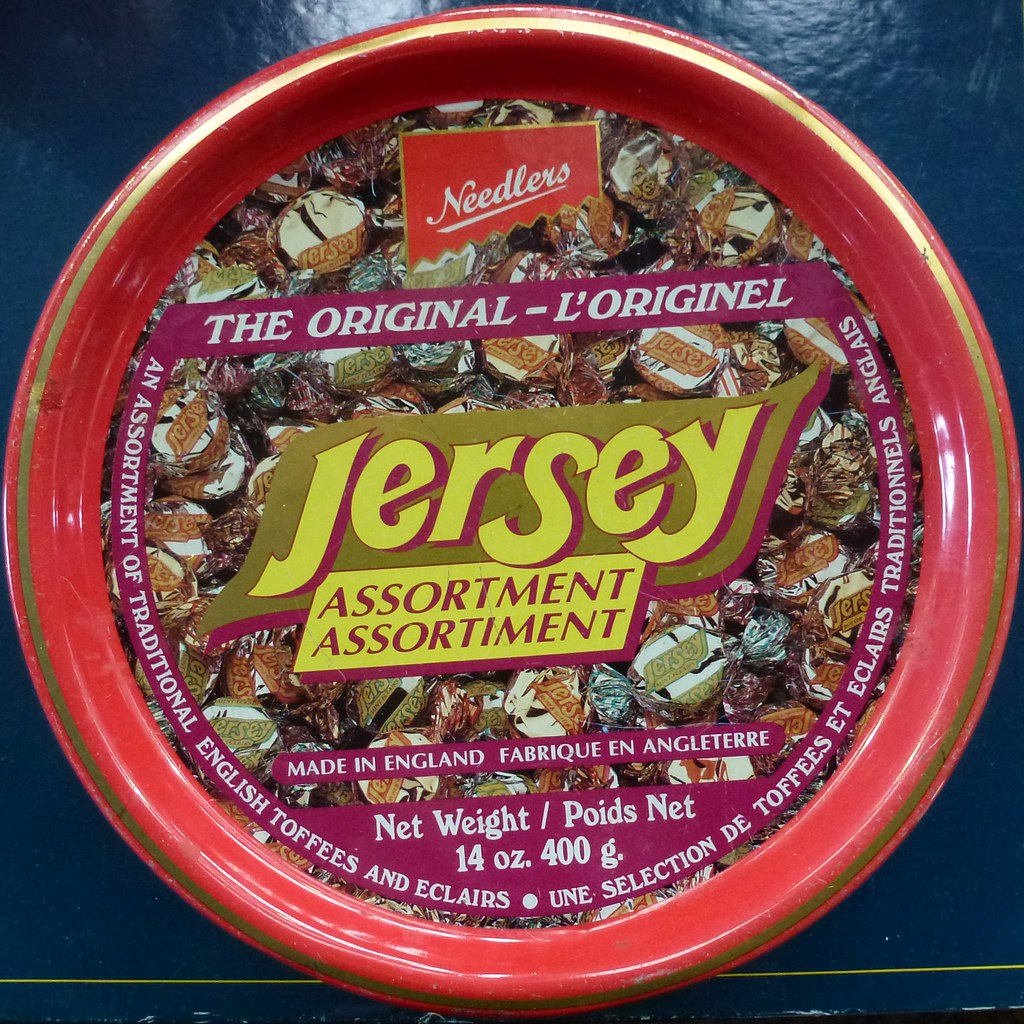The image captures a detailed top view of a circular red tin container made for food, specifically an assortment of traditional English toffees and eclairs. The tin prominently features a Needlers logo in white cursive font on a red background positioned at the top. Below this, the label reads "The Original" in white text on a purple background, followed by "Jersey Assortment" in yellow text with a goldish background. Surrounding the central logo, the tin displays gold-wrapped candies with the Jersey logo on them. The text also includes bilingual labeling, with phrases like "Made in England" and its French translation "Fabriqué en Angleterre." The net weight is indicated as 14 ounces (400 grams). The background of the label and container is a combination of purple and red, with the candy wrappers creating a metallic, festive appearance. The overall backdrop of the image appears to be a dark blue surface.